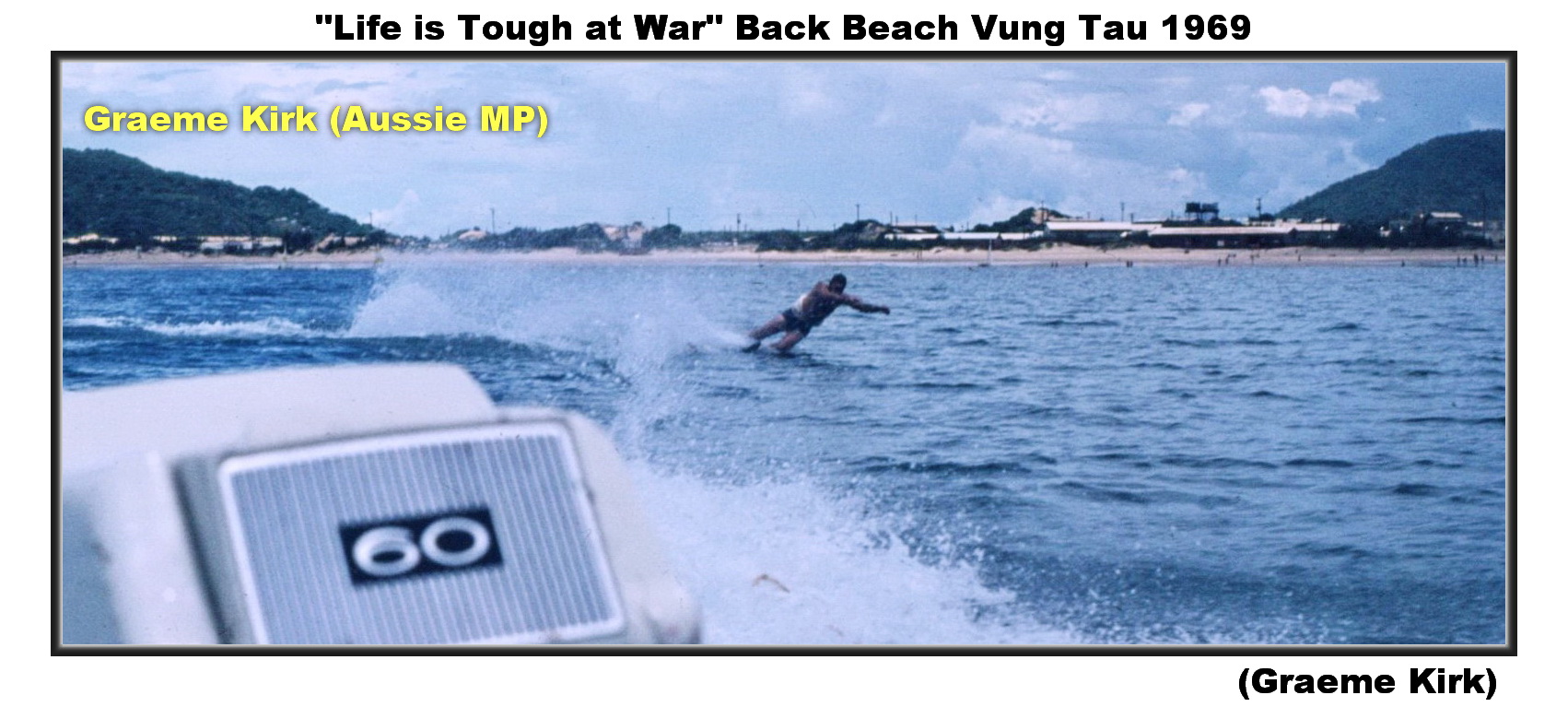This rectangular, old-looking photograph with a faded blue tint depicts a man struggling to maintain balance while water skiing on a body of water, likely pulled by a boat. The boat's white motor, labeled with the number "60," is visible on the bottom left. Above the photograph, the words "Life is Tough at War" are printed in black within a black border, centered on a white background. The top left corner of the image features yellow text reading "Graeme Kirk, Aussie MP," while the same name, "Graeme Kirk," reappears in black on the bottom right. In the background, a coastline with sandy beaches, a few buildings, and faint mountain ranges under a blue and white sky can be seen. The scene is set at Back Beach, Vung Tau, Vietnam, in 1969.